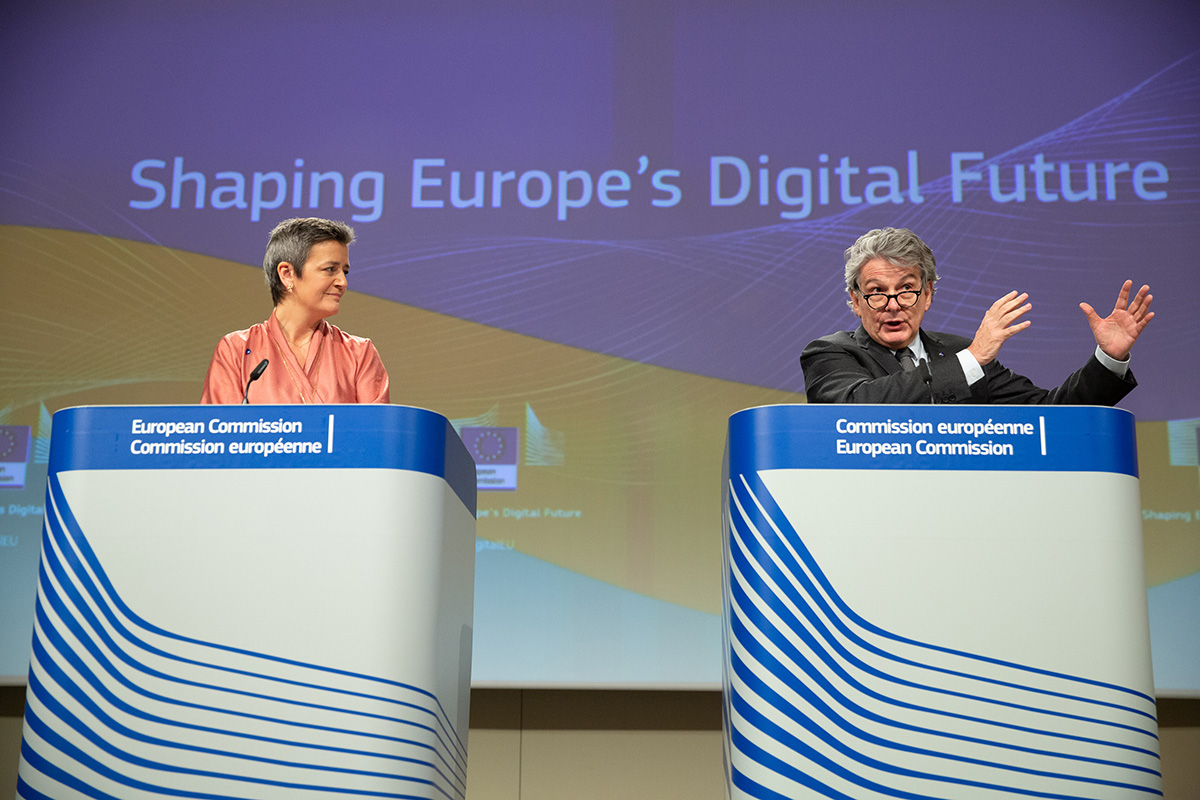In the image, a color photo, the backdrop displays a large sign with the text "Shaping Europe's Digital Future" in prominent blue letters. This background comprises a mix of purple, tan, and white diagonal blocks interspersed with wavy white designs reminiscent of digital imagery. The setting features two curved white lecterns with blue trim at the top, each labele' "European Commission" and "Commission Européenne." To the left, a woman with short salt-and-pepper hair stands at one lectern, dressed in a coral pink blouse and small earrings. She appears to be around 40-50 years old, intently looking at the man beside her. On the right, the man, who has salt-and-pepper hair and wears black wireframe glasses, is dressed in a black suit, white shirt, and a dark tie. He is actively gesticulating and speaking, addressing the audience with a professorial demeanor. Both speakers have small microphones mounted on their lecterns, indicating they are engaged in delivering an important lecture or debate.